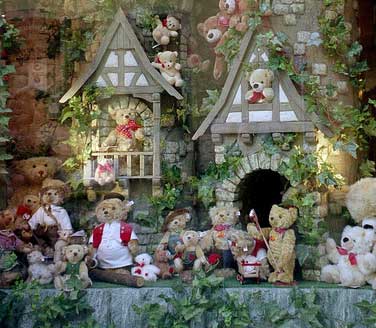This image showcases an elaborate and detailed display of various stuffed teddy bears set against a backdrop resembling a miniature castle or house with multiple towers and windows. The scene is intricately designed with grayish rock ground, and the beige and light brown structures feature small cave-like enclosures. Green ivy vines with lush leaves climb up the walls, enhancing the whimsical atmosphere. The teddy bears are diverse in size, shape, and appearance, predominantly brown, with some white ones, and a few adorned with reddish ribbons or clothes. Many of the bears are positioned at the windows, looking outwards, while others are strategically placed around the buildings, creating a charming and lively scene.